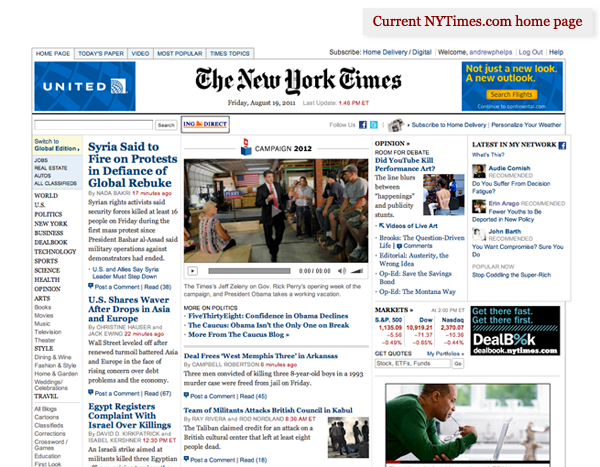A digital screenshot of the New York Times homepage from Friday, August 29th, 2011, displaying various interactive sections that mimic its print version. At the top left-hand corner, the 'Home' page is highlighted, indicating the current view. Adjacent links include 'Today's Paper,' 'Video,' 'Most Popular,' and 'Times Topics.' On the right side, options for 'Subscribe'—offering home delivery or digital—are visible. A welcome message addressed to Andrew Phelps appears next, followed by links to 'Log Out' and 'Help.' A red header announces 'Current NYTimes.com Home Page.' Further down, the layout resembles a traditional newspaper, featuring written articles, some accompanied by images, sections displaying stock market figures, and various advertisements. On the left side, there are links to other sections such as 'Global Edition,' 'Jobs,' 'Real Estate,' 'Autos,' and 'Classifieds,' providing a comprehensive digital reading experience.